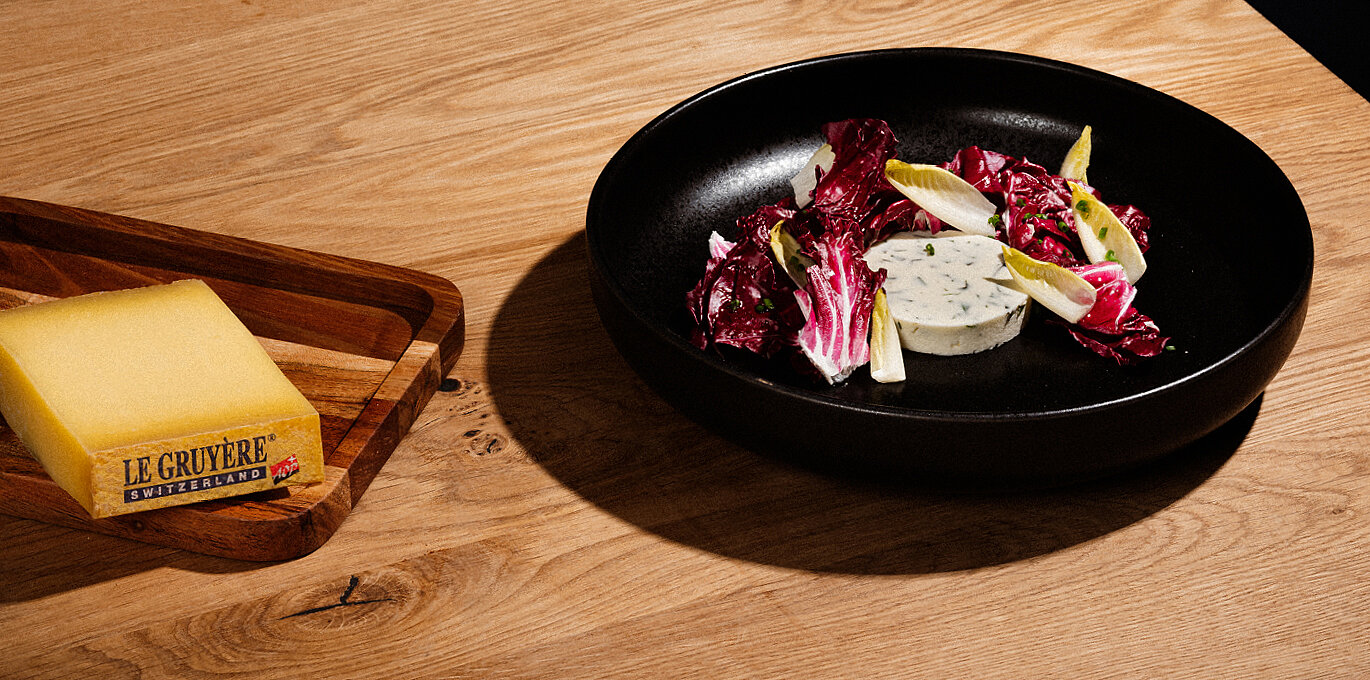The image depicts a sophisticated food presentation set on a light, unvarnished wooden table with visible wood grain. Centrally positioned is a shiny, black stainless steel pan of a large circular shape. Inside the pan, an herbed butter circle or possibly a piece of cheese sits in the center, surrounded by a colorful assortment of purple, pink, and yellow salad leaves. Adjacent to the pan, on the left, is a walnut cutting board showcasing a block of Le Gruyere cheese from Switzerland, prominently labeled. The arrangement is lit from the right side, casting shadows to the left, and part of the black background is visible in the upper right corner, framing the elegant setup.